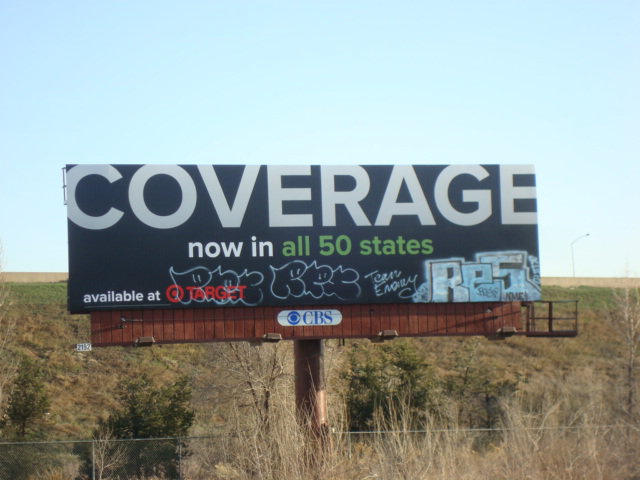The photograph captures a billboard situated outdoors, mounted on a vertically erected brown cylinder post. The post leads up to a brown metal railing and rests on a brown vertical wood-paneled base. The billboard itself is predominantly black with white text that reads "COVERAGE, now in all 50 states," where the phrase "all 50 states" stands out in green. On the bottom left corner, the text "AVAILABLE AT TARGET" is accompanied by the familiar Target Bullseye logo. 

The CBS logo, a simple white design set against a blue background, is also present, though its exact placement on the billboard isn't specified.

There is a layer of graffiti in white lettering, seemingly spelling out "RE5" in a blue and white blocky style, although the exact message is unclear. The base of the billboard is surrounded by a patch of overgrown brown grass, while a clear blue sky forms the backdrop, highlighting the billboard and its surroundings.